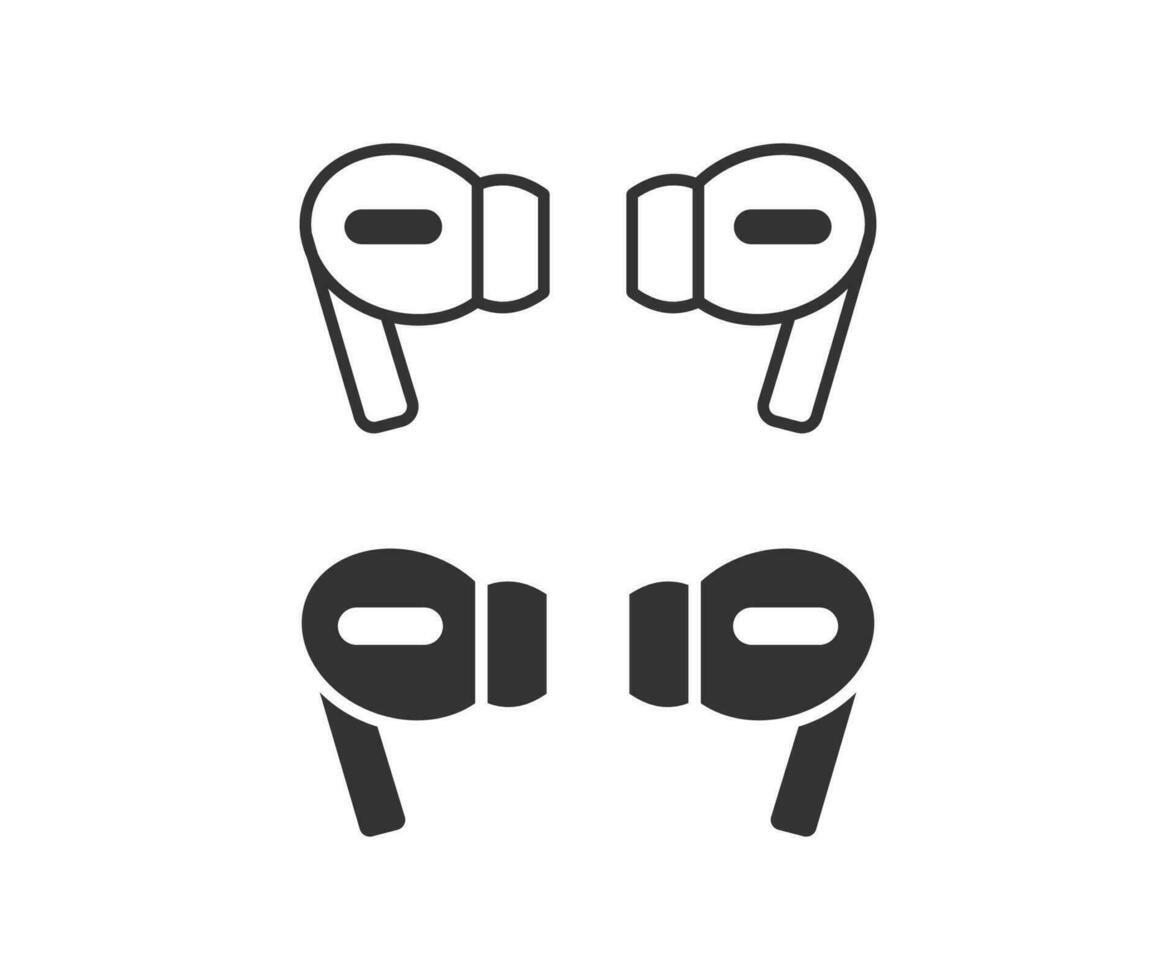This image features a white background displaying four earbuds arranged in a 2x2 grid. In the top row, there are two predominantly white earbuds outlined in black, each featuring a small black oval near the center. These earbuds are positioned to face each other, with a slight gap separating them. Similarly, the bottom row showcases two predominantly black earbuds, mirroring the top row’s layout by also facing each other with a small central gap. Both sets of earbuds create the visual illusion reminiscent of eyeglasses split down the middle. Each earbud is approximately three-quarters of an inch in height and width, and the entire image measures around three inches squared.